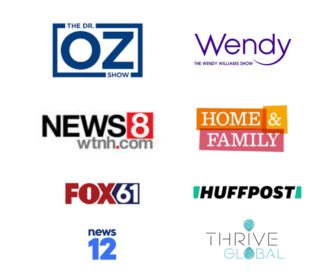The image displays a screenshot divided into eight distinct segments, each representing a TV show or news channel. The layout consists of two columns, each containing four blocks.

In the first column (from top to bottom):
1. **The Dr. Oz Show**: Dominated by the prominent word "Oz" centered within a rectangle, with "The Dr." and "Show" in smaller fonts at the top and bottom, respectively.
2. **News 8**: Features the text "News 8" prominently, accompanied by the URL "WTNH.com." Notably, the dot in the URL is red, and the number 8 is enclosed within a red box.
3. **Fox 61**: The channel's logo showcases the number 61 in white set against a navy blue background.
4. **News 12**: This segment has a blue background with the text "News 12."

In the second column (from top to bottom):
1. **The Wendy Williams Show**: Emphasizes the name "Wendy" at the top.
2. **Home and Family**: Displays the title "Home and Family."
3. **Huff Post**: Simply labeled "Huff Post."
4. **Thrive Global**: Displays the name "Thrive Global."

Each block is visually distinct, reflecting the branding elements typical of their respective shows or channels.